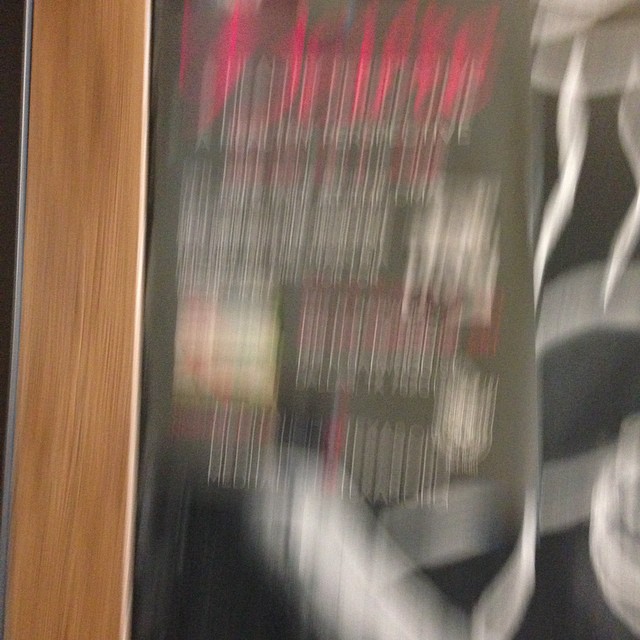The image is a very blurry photograph, possibly of an advertisement or menu. On the left side, there is a visible medium brown wooden plank or slab, which may be the side of a door or wall. The center of the image is dominated by a blurry menu or sign. The upper part has indistinguishable red or neon pink text that fades into white lines. There are small, indistinct drawings or decorations on the menu. To the right, there are thick, silver, ribbon-like objects intertwined and hanging down, seemingly from the ceiling. The background is a gray color with random flowy white objects scattered throughout. The leftmost part next to the wooden plank is a plain dark black.